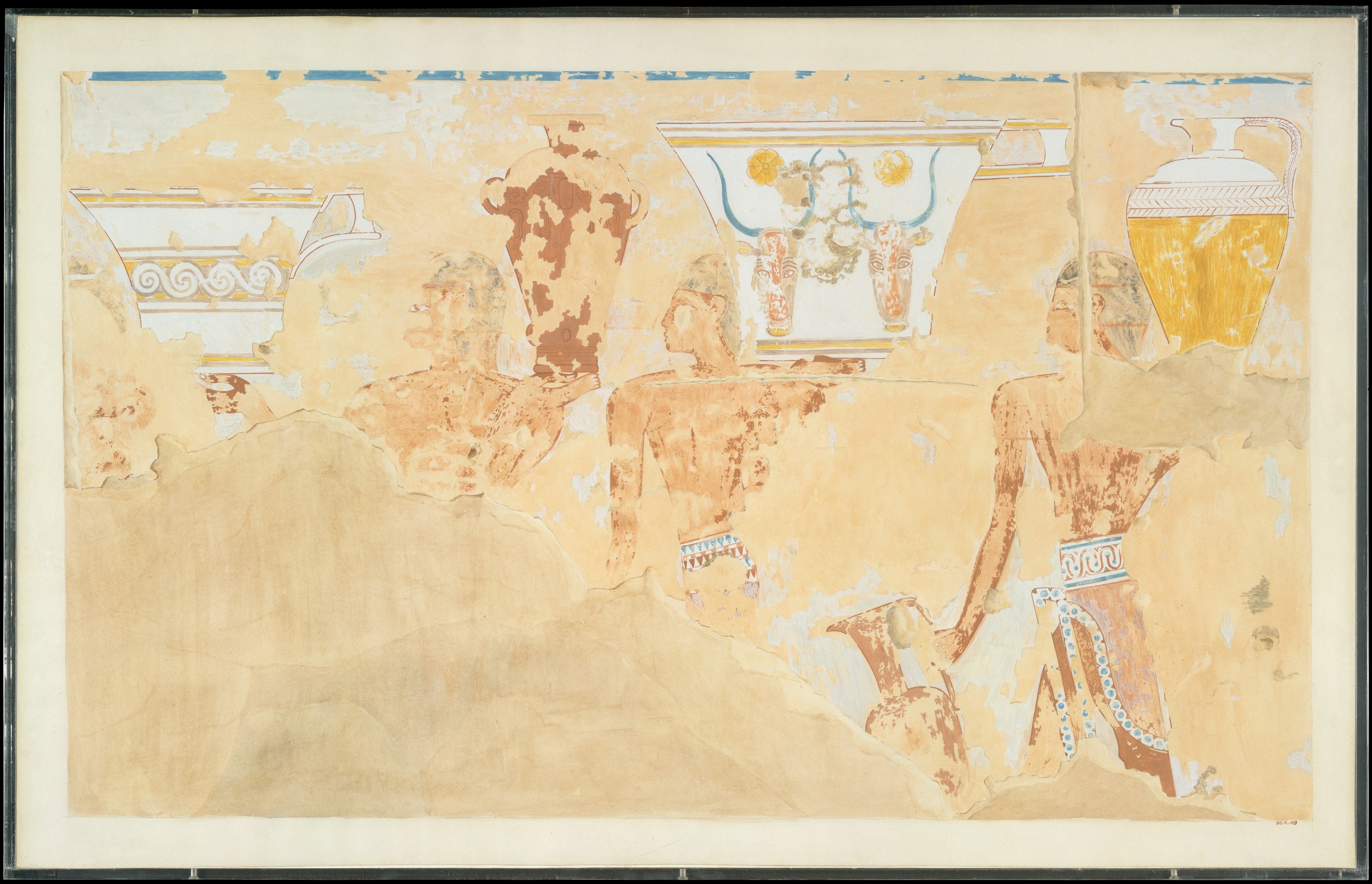This image is a distressed and worn painting in the Egyptian style, featuring a line of at least three figures carrying ornate urns and pitchers. The figures are clad in traditional sarongs, emphasizing their Egyptian association. The painting shows signs of significant wear, particularly in the bottom left-hand corner, where it appears the paint has chipped away or been ruined over time, obscuring some details. The figures, whose faces lack detail due to the aging of the artwork, are depicted in a procession starting from the right front corner and moving towards the left. The individual at the back, most clearly visible, carries a large urn on their right shoulder and a smaller one in their left hand. The next figure also bears a large container decorated with what seems to be images of bulls' heads. The painting is richly intricate in the design of the vases, although much of the color and detail has faded, adding to its aura of antiquity and authenticity.